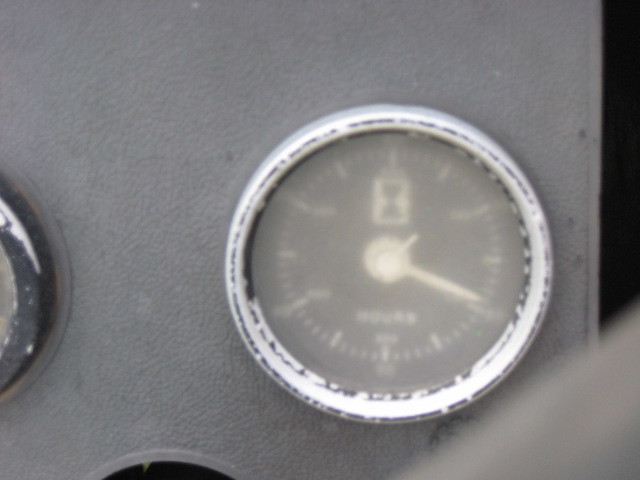This horizontal rectangular photograph, set against a gray wall, features a vintage clock as its central subject. The clock has an outer circular ring that is predominantly white, although it is worn in places, revealing spots of rust or exposed iron. The clock face lacks traditional numerals, instead displaying lines to mark the hours. Both the clock hands and the lines appear to be a cream or light yellow color, although the image is slightly blurry, making finer details difficult to discern.

In the bottom right corner of the image is a small, blurred feature. Additionally, there is a partially visible round object with a shiny surface on the middle left side of the photograph, along with a hint of another rounded dome-like object at the bottom left. The rightmost quarter of the photograph is marked by a thick, black horizontal area, adding contrast to the composition. The overall image evokes a sense of antiquity and wear, enhanced by the visible imperfections and muted color scheme.